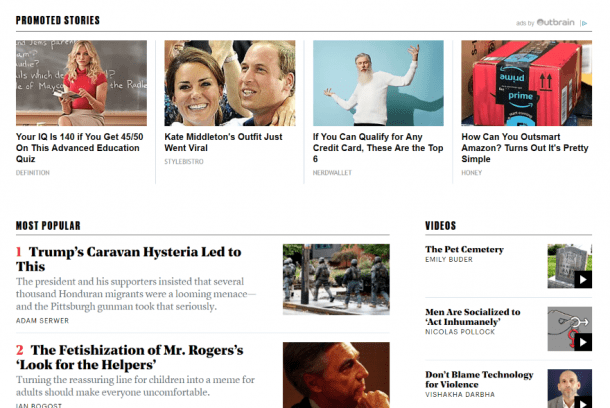Here is the cleaned-up and detailed caption:

---

This is a screenshot from a news or magazine website, known for featuring clickbait articles. The background is primarily white, and the page is headed by the label "Promoted Stories" in the top left corner, indicating the content is likely sponsored. Below this heading, four images are arranged horizontally with their corresponding provocative headlines.

Starting from the left:

1. An image of a provocatively-dressed blonde woman sitting on a teacher’s desk in front of a blackboard. The accompanying headline reads, “Your IQ is 140 if you get 45/50 on this advanced education quiz.”
2. A photo capturing Prince Charles and Kate Middleton smiling and embracing. The related headline states, “Kate Middleton’s outfit just went viral.”
3. A picture of an older man with a white beard and wearing a white, long-sleeved t-shirt, standing against a blue background. The text below this image reads, “If you can qualify for any credit card, these are the top six.”
4. An image of a standard Amazon Prime package, identifiable by its black tape with blue Amazon Prime branding. The headline beneath it asks, “How can you outsmart Amazon? Turns out it’s pretty simple.”

Each of these stories uses attention-grabbing visuals and intriguing headlines to entice readers to click.